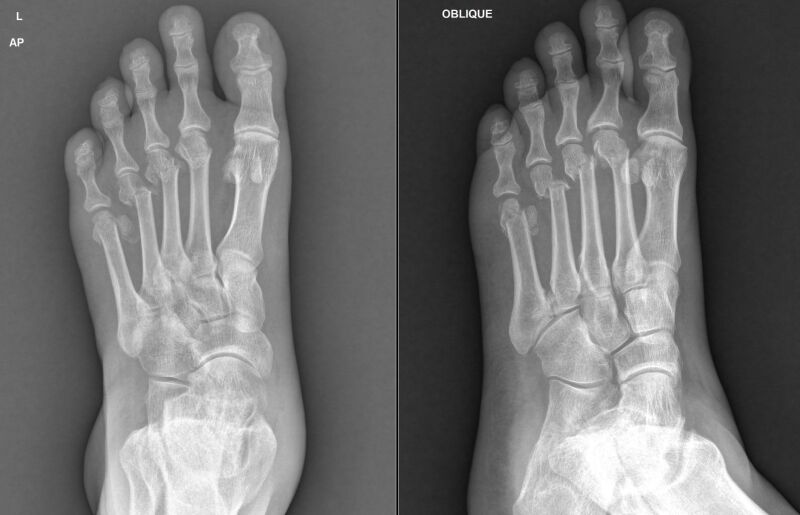This image is a rectangular x-ray diptych, approximately six inches wide and three inches high, displaying two views of the left foot. The left x-ray has a lighter gray background and is labeled with a white "L" and "AP" in the upper left corner. It shows a top-down view of the foot, from ankle to toes, revealing fractures across the metatarsals before the toe area. The right x-ray has a darker gray background, also in the upper left corner, labeled "oblique." This side-view image shows the foot slightly turned on its side, enhancing visibility of the fractures. At least four bones appear completely displaced near the knuckle areas.